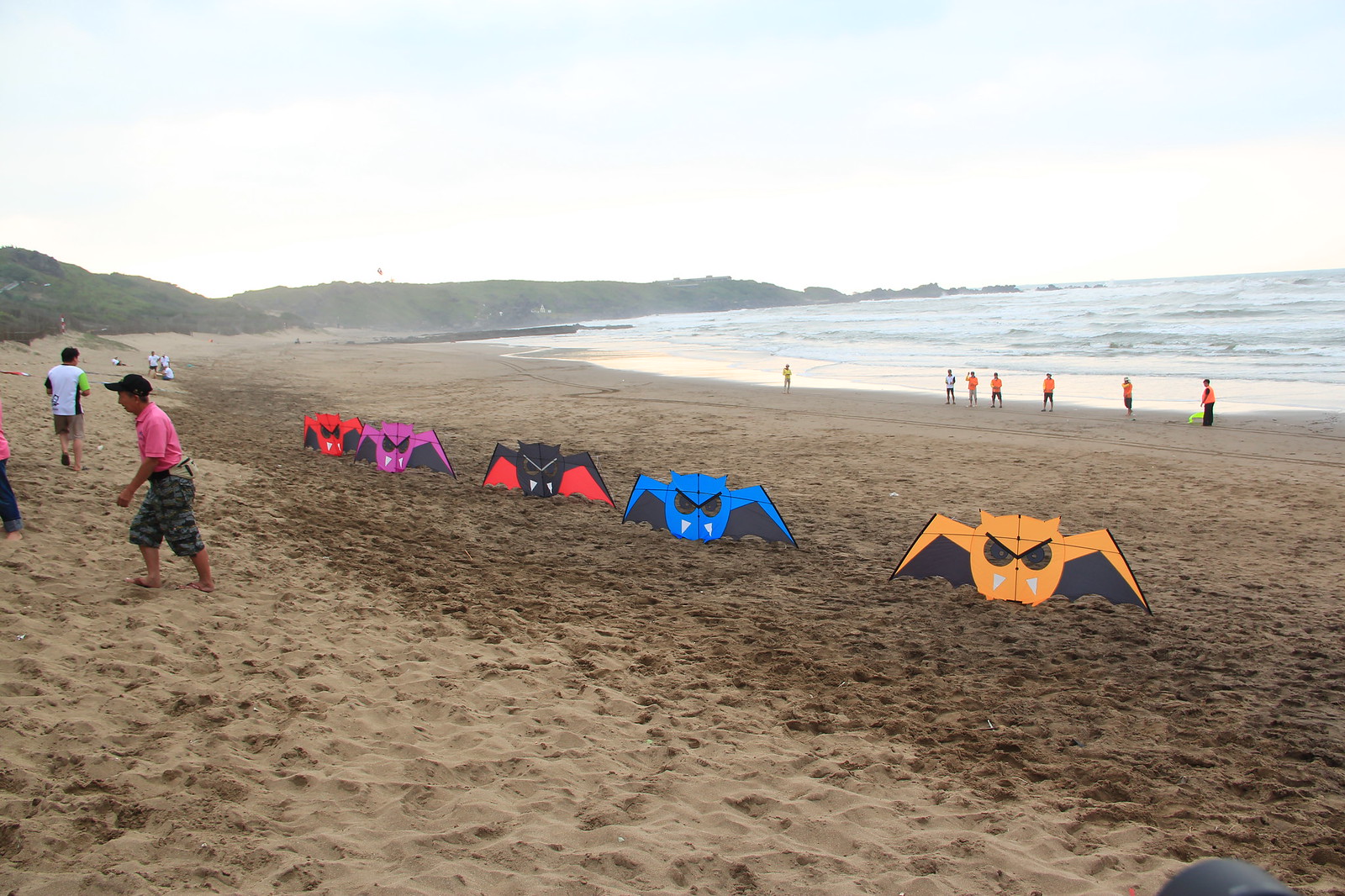A sprawling beach stretches across the foreground, with lighter sand giving way to darker sand near the water's edge. Scattered footprints mark the sand where several people are walking, including a man in a pink shirt and cargo shorts, and another in a white shirt. Near the coastline, six individuals in orange shirts and one in white appear to be organizing an event. Alongside the water, five colorful kite-like structures resembling bats stand on display. These structures feature black eyes and fangs, and are colored orange, blue, red, purple, and another shade of blue, giving them a frowning appearance. In the background, green hills and mounds of dirt rise up under a white sky, completing the scenic view.